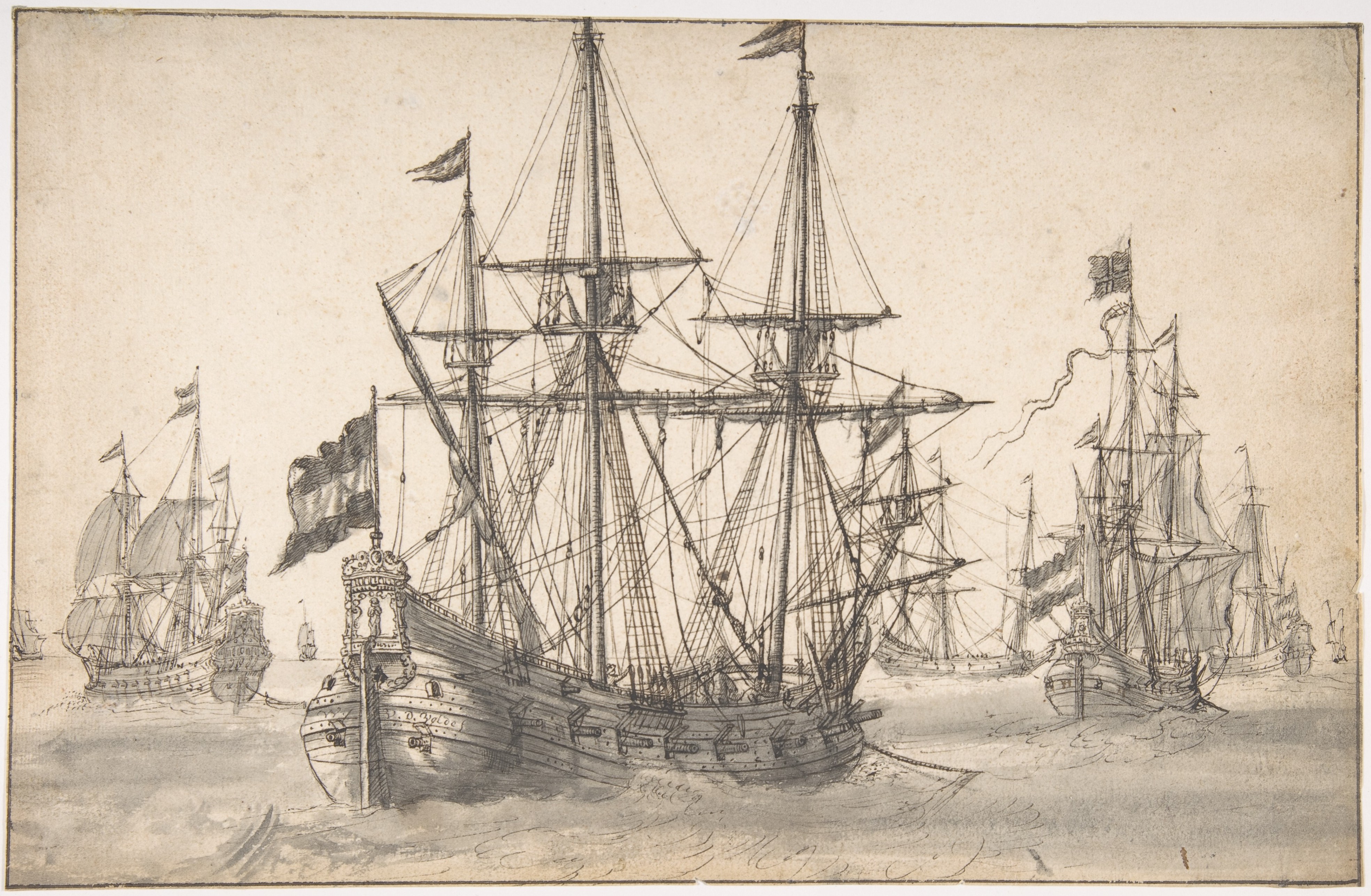This pencil drawing depicts a serene water scene with seven intricately detailed wooden ships. Each ship is crafted meticulously from wooden planks and is equipped with large masts intertwined with what seems like hundreds of ropes. The prominent ship in the foreground lacks sails but is adorned with a distinctive flag at its stern, featuring alternating dark and light stripes. Surrounding this ship are several others, their voluminous sails billowing robustly in the wind. Cannons jut out from the sides of the main ship, adding a historical touch, while smaller flags flutter atop the masts, capturing the essence of an era long past. The entire scene is skillfully rendered, showcasing the artist’s attention to detail and mastery of pencil work.